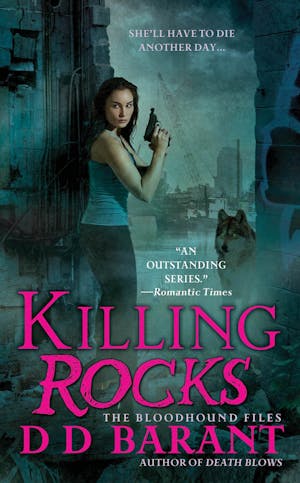The cover of the book "Killing Rocks," part of "The Bloodhound Files," by D.D. Barant, features a vibrant, full-color image. Dominating the cover is a young Caucasian woman with dark hair, dressed in a blue tank top and black pants. She holds a black pistol in a defensive posture and is standing in a stone doorway. Her body faces right, but she looks over her shoulder to the left. To her right, a ghostly wolf stands sentinel, with a cityscape visible through its transparent form in the background. The city includes a body of water, a ship, a tugboat, and several tall buildings. The title, "Killing Rocks," is prominently displayed in bold pink text, while above it, a white text review from Romantic Times reads, "An Outstanding Series." Additional white text at the top declares, "She'll have to die another day," branding the novel as part of a thrilling narrative. The author's name, D.D. Barant, is noted as the writer of "Death Blows."